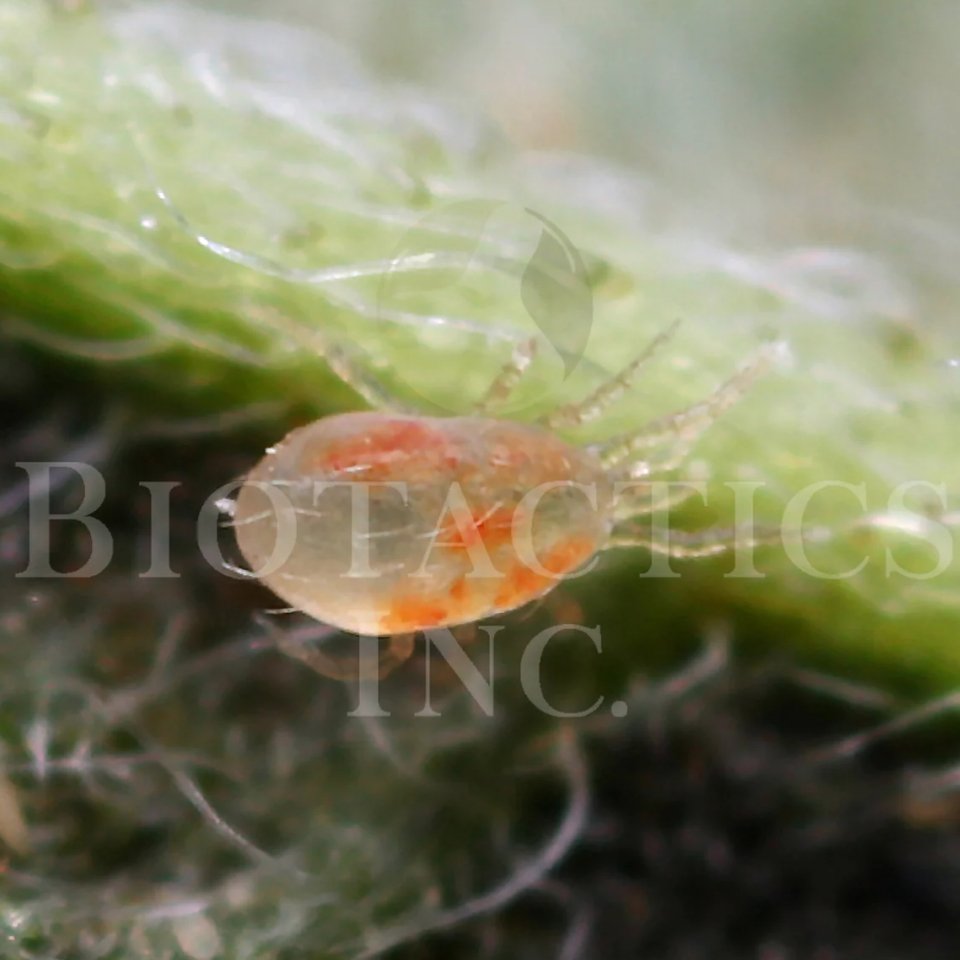In the center of the image, there is a semi-translucent, oblong creature measuring roughly over an inch wide and three-quarters of an inch high. The creature features a clear, gel-like body with multiple orange spots, possibly indicating internal organs. It appears to have segments or tentacle-like appendages extending from it, including eight semi-transparent legs and two small pincers to the right. This looks like a microscopic sea organism or possibly an octopus or squid larvae. The background is blurred, highlighting a light green plant adorned with fine, white threads or vines. The photograph is outdoors and slightly blurry overall, but clear enough to make out the main subject. Across the center of the image, in a faded, transparent white text, it reads "Biotactics Inc."